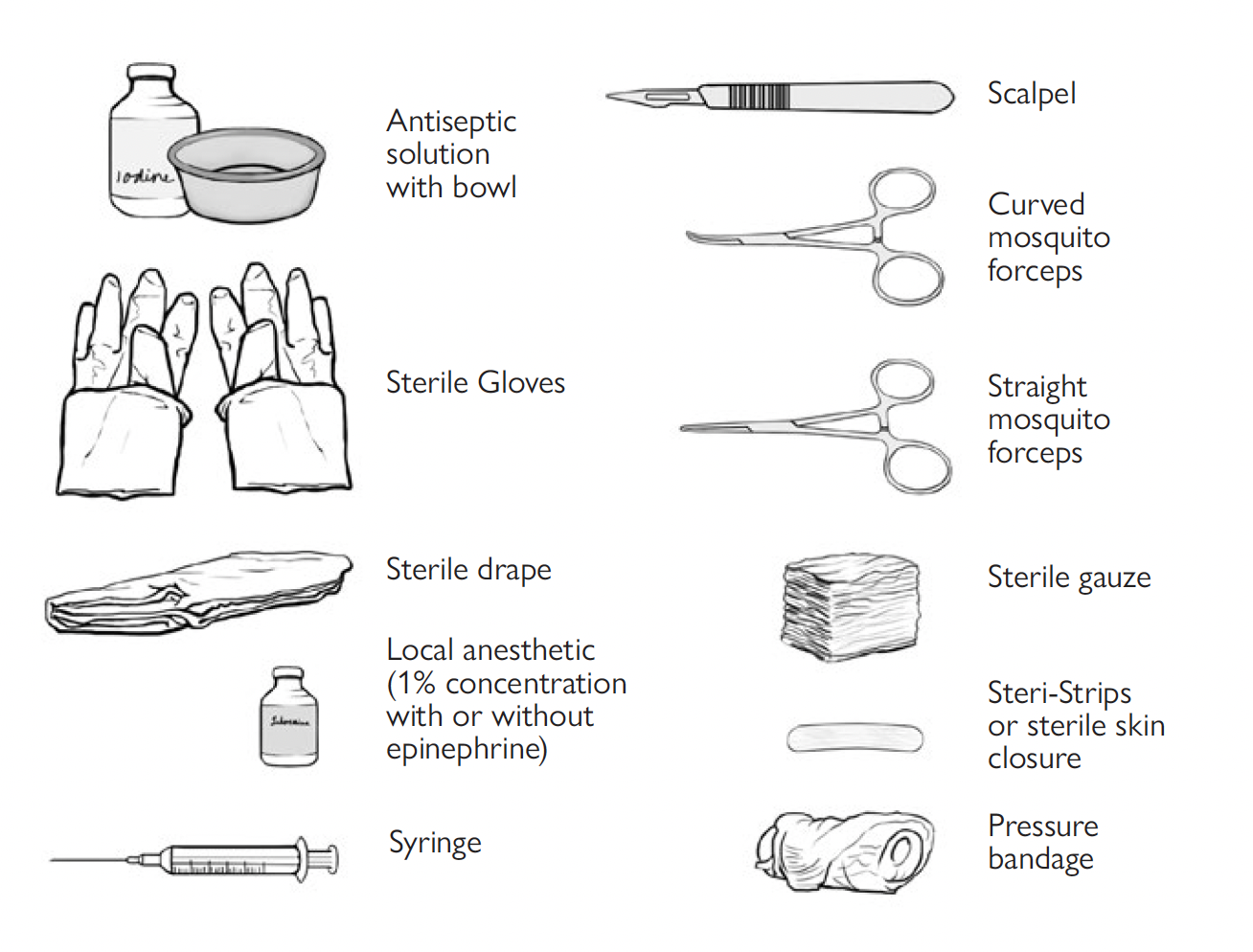This black and white illustrated diagram meticulously details an array of essential medical instruments, neatly organized into two columns. On the left column, from top to bottom, there are drawings labeled "Antiseptic Solution with Bowl" featuring a bottle marked "Iodine" next to a small bowl, followed by "Sterile Gloves" resembling disposable gloves, then "Sterile Drape" depicted as a folded towel, and "Local Anesthetic (1% concentration with or without epinephrine)" shown as a small glass bottle, concluding with a standard "Syringe" with a needle. The right column starts with a "Scalpel," followed by "Curved Mosquito Forceps" and "Straight Mosquito Forceps," both portrayed as forceps with one having a curved tip and the other straight, next is "Sterile Gauze" packaged in a stack, continuing with "Sterile Strips or Sterile Skin Closure" meant for wound closure, and ending with a "Pressure Bandage," illustrated as a roll of flexible adhesive wrap similar to vet wrap. This detailed depiction emphasizes the organized structure and comprehensive labeling of each medical tool.